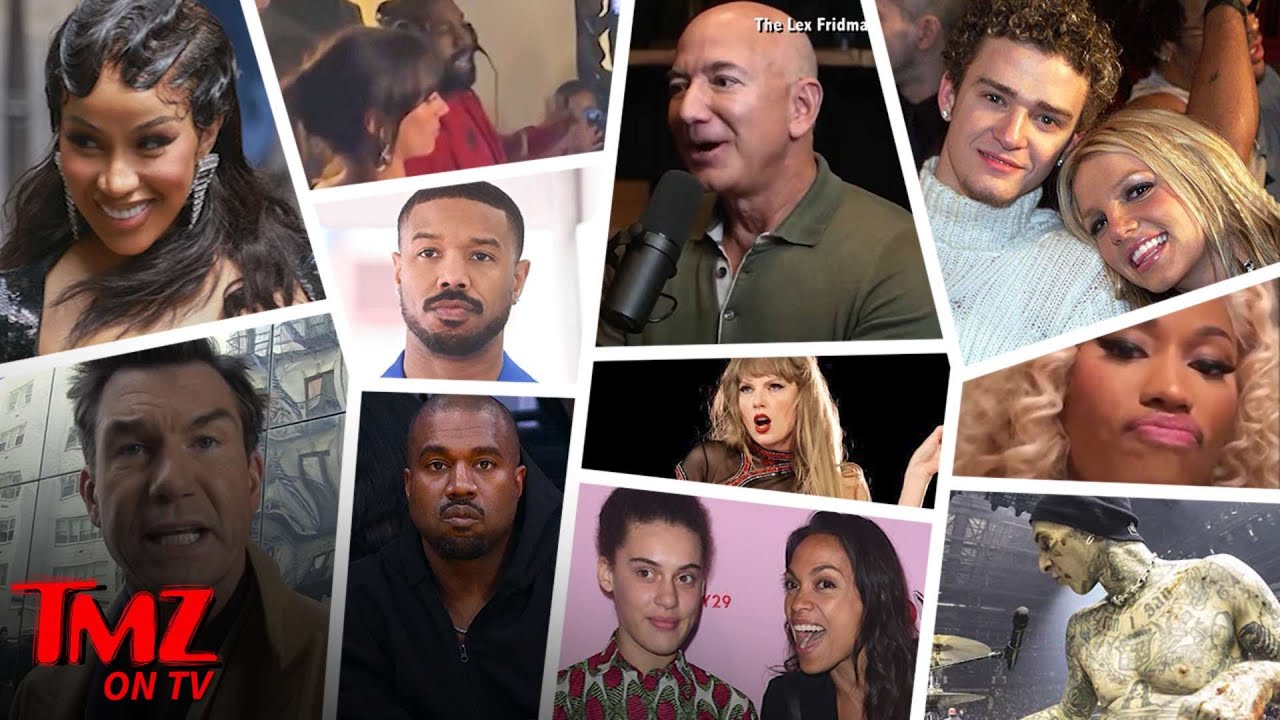This image is a TMZ collage featuring numerous celebrities. In the bottom left corner, the TMZ logo is visible, reading "TMZ on TV." Another piece of text, possibly a copyright trademark, is positioned near the middle top, slightly to the right, with the "Lex Freed Min" part cropped out. 

The collage predominantly consists of paparazzi photos, though some may be promotional shots. Starting from the top left, there is an image of Cardi B. The bottom left includes another actor. The collage also features business magnate Jeff Bezos among a variety of personalities, mostly musicians and actors.

Notable among the musicians are Justin Timberlake and Britney Spears, seen in a vintage photo from their dating days. Additionally, the collage includes images of Nicki Minaj, Taylor Swift, and Kanye West. From the rock genre, Travis Barker, drummer from Blink-182, is also depicted. The collage showcases several other celebrities as well, offering a snapshot of diverse and prominent figures in the entertainment and business worlds.